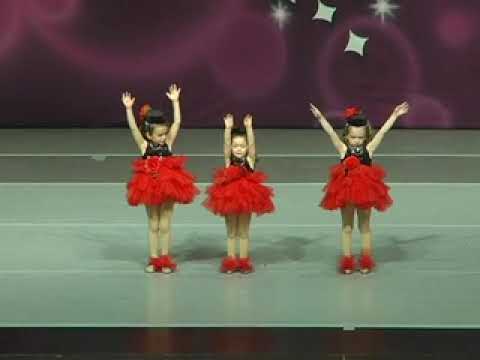The image depicts a grainy still from a home recording of a performance featuring three young girls, likely around nine or ten years old, on a stage. Their attire includes red and black accessories in their hair, possibly bows or hats, black jumpers paired with red frilly tutus, and red shoes or slippers. The stage itself is marked by bands of enamel gray lines, comprising three lighter lines and two darker lines. In the background, there's a purple screen adorned with pink circles and displaying the stylized text "Rainbow Connection," with the 'R' designed to resemble a dancer executing a split leap. The girls on stage are engaged in a synchronized routine, each with their hands raised, set against this vivid backdrop. Additionally, a black rectangle is visible at the bottom of the photo, possibly framing the image.